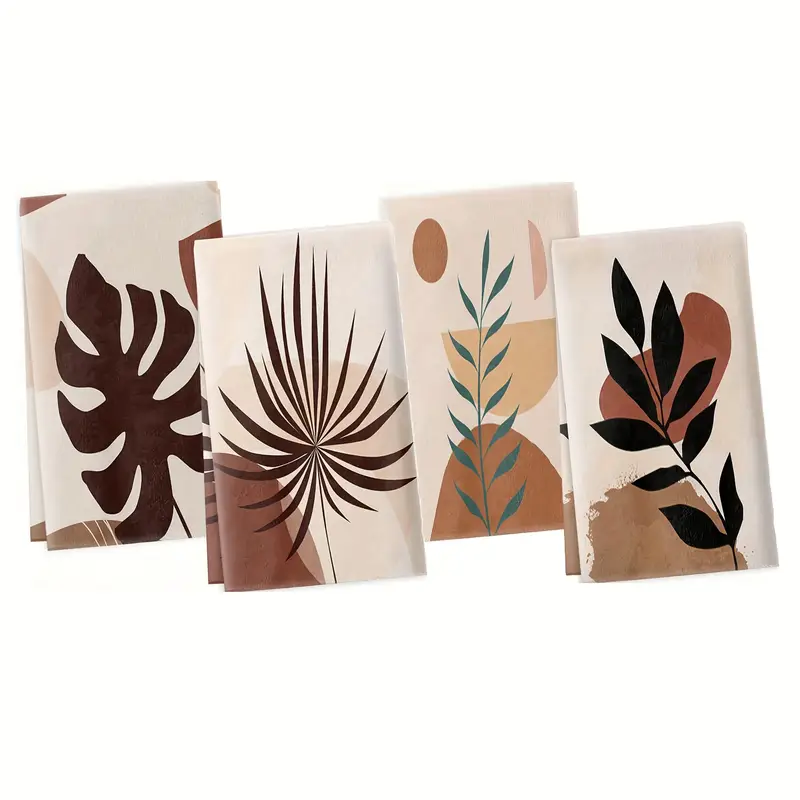The image displays four folded cloth napkins, arranged side-by-side with slight overlapping, against an absent background. Each napkin is intricately designed and folded into a rectangular shape suitable for a table setting. The first napkin on the left features a brown Monstera plant print on a light tan background, complemented by additional brown and cream decorations. The second napkin also has a tan background and displays a brown palm plant motif with similar brown accents. The third napkin showcases a long green fern surrounded by half-moon and circular patterns. Finally, the fourth napkin presents a black illustration of a plant with wide black leaves that cover brown decorations on a beige tan background. The designs on these napkins incorporate abstract plant imagery in various earthy tones and illustrate a combination of natural forms with stylized decorative elements.